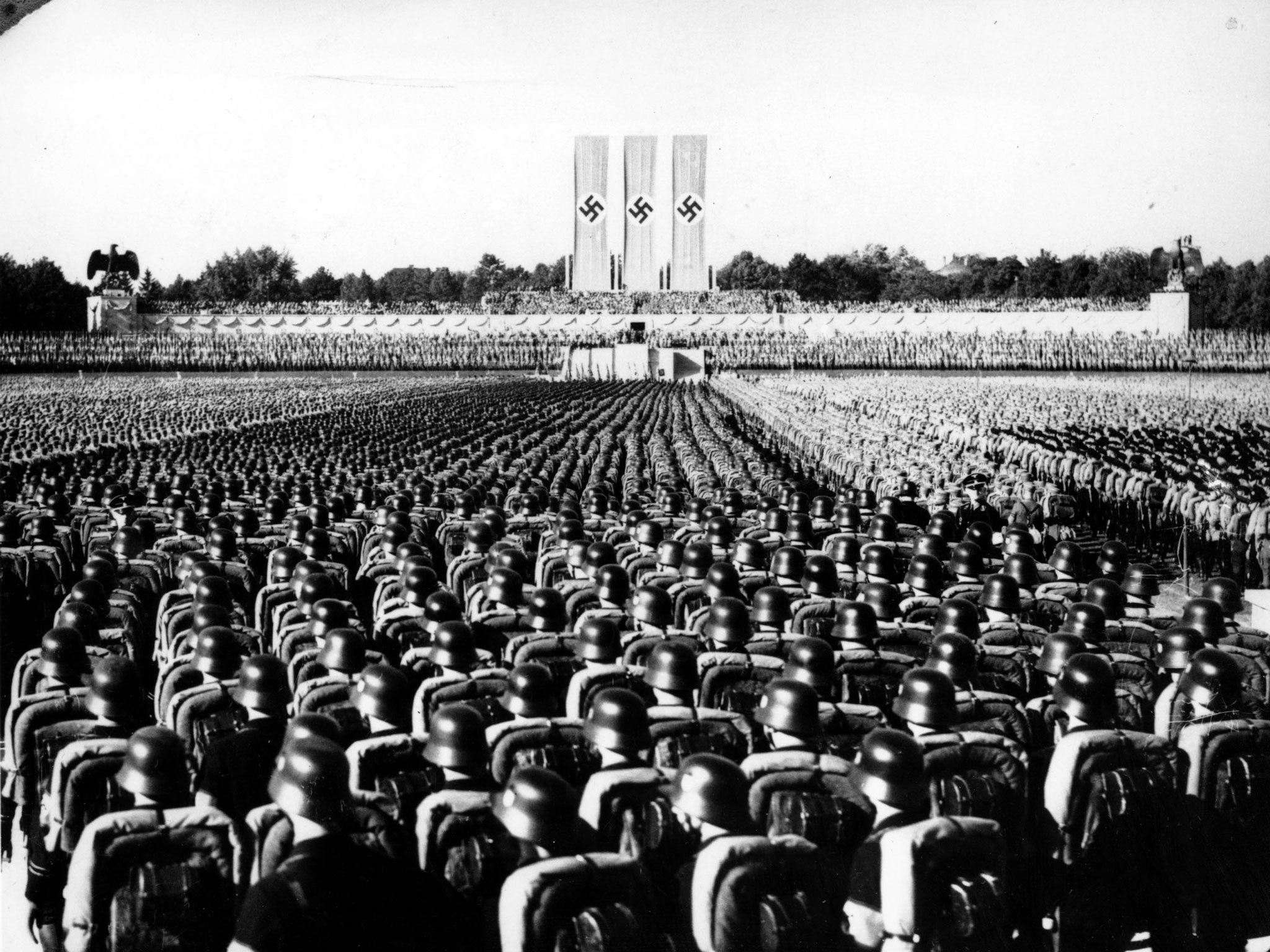This is a highly detailed black and white drawing styled to mimic a photograph, potentially an actual photograph. Dominating the foreground, thousands of Nazi soldiers stand shoulder to shoulder, their backs turned towards the viewer, all donning rounded helmets and rectangular backpacks. The immense crowd fills nearly the entire frame. 

In the middle ground, they collectively face a grand stand or podium, which is composed of five rectangular sections with the tallest in the center. Towering over this podium are three large vertical banners or silo-like structures, each emblazoned with a distinctive Nazi swastika set in a black circle on a white background. To the left of these structures, a prominent eagle statue and a row of trees add additional features to the solemn scene. The sky above is an overcast gray, void of clouds, emphasizing the monochrome and somber tone of the image.